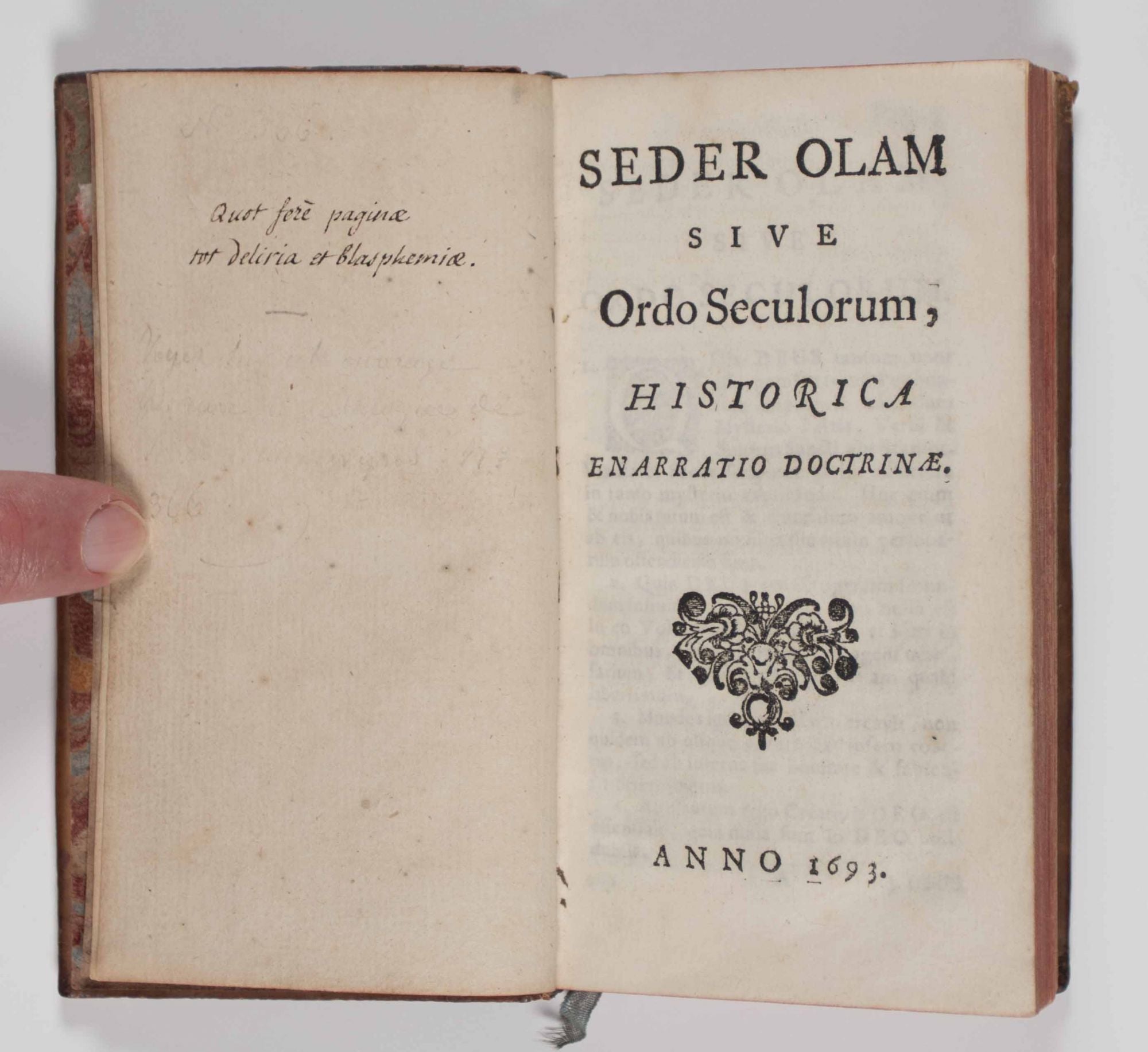The image captures an aged, hard-backed book opened to what appears to be the front page or possibly the second page, given its positioning. The language used is not English, with text that reads "Quant forae pagine tot deliria of blasphonice" and on the adjoining page, "Cedar alam sive ordo secularium historica annarato doctrine." The bottom of the right page states "Anno 1693," indicating its year of publication. The book's pages show significant aging, with faded colors and a reddish tone along the edges. A slightly jagged index finger of a person of Caucasian descent, positioned towards the left side of the book, is holding the page open. The image itself is square, approximately six inches by six inches, with a light gray border or background, likely indicating it is resting on a surface. A distinct stamp or emblem featuring floral designs and horses' heads is present, suggesting a publisher's mark or perhaps a national emblem from the late 17th century.